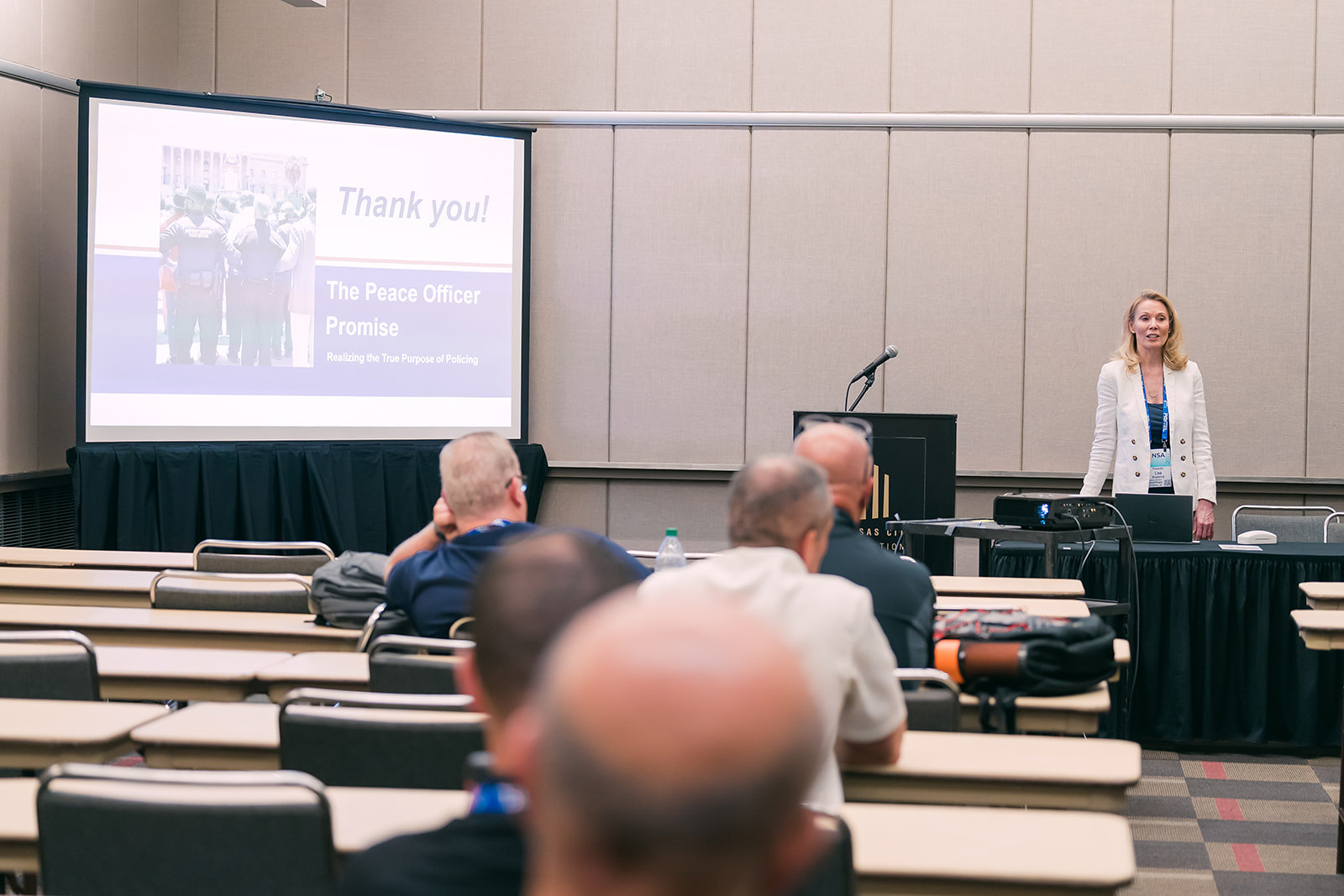In the image, we see a detailed scene of a presentation taking place in a cream-colored conference room with a pattern of vertical rectangles and horizontal white bars. A middle-aged woman with blonde, shoulder-length hair, wearing a white blazer over a blue shirt and an ID card hanging around her neck, is seated at the front behind a table draped with a black tablecloth. On the table, there is a laptop and a projector. To her right stands a podium with a silver microphone and an unreadable logo. The projector displays an image on the screen in the corner of the room, showing a text that reads, "Thank you, the peace officer promise," along with a picture of peace officers.

In front of her, there are six men—most with balding heads, suggesting they are older—seated at brown tables with black chairs, their backs turned towards the camera. They appear to be attentively listening to the presentation. Some have backpacks and water bottles on the tables in front of them, and the room gives off an organized, formal atmosphere common in professional or academic settings.